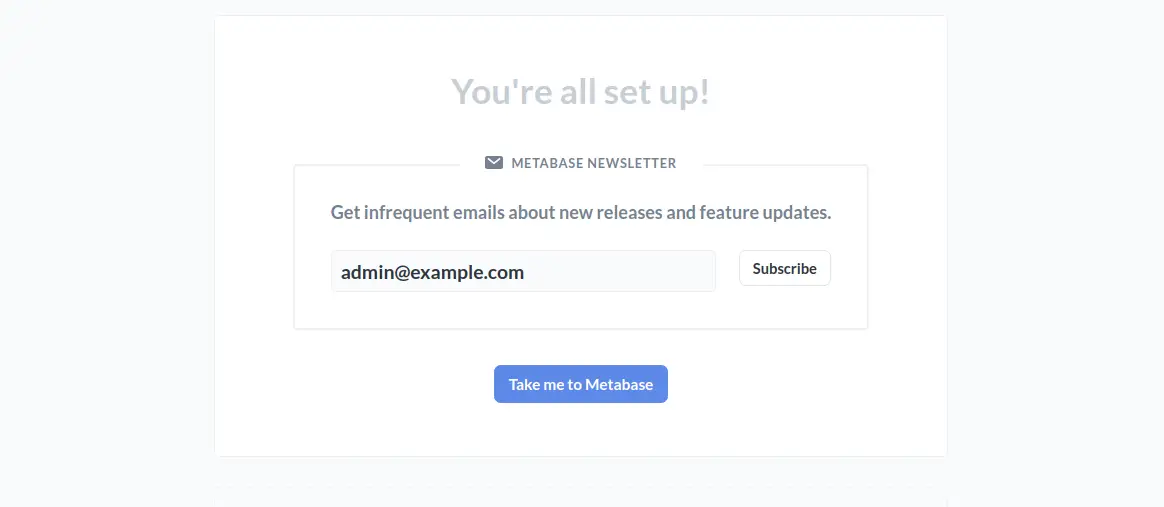The image captures the confirmation page of a newsletter sign-up, likely for the MetaVase Newsletter. The focal point of the page is the bold, capitalized, light gray text at the top that reads, "YOU'RE ALL SET UP." Directly beneath this message, there's a dark gray icon featuring an envelope, accompanied by the text "MetaVase Newsletter."

The page's background contains a subtle message that states, "Get infrequent email about new releases and future updates." Just below this message, on the left side of the image, appears an email address formatted as admin@example.com in bold, dark text, indicating this as a placeholder or example email within the input box. On the right side, the word "Subscribe" is present.

At the lower part of the overlay, there's a blue rectangle button labeled, "Take me to MetaVase," with white text and a capital 'M'. The entire layout is housed within a white square box, which has a faint border. The backdrop of the page features lighter shades of blue and gray, adding a soft contrast to the overall design.